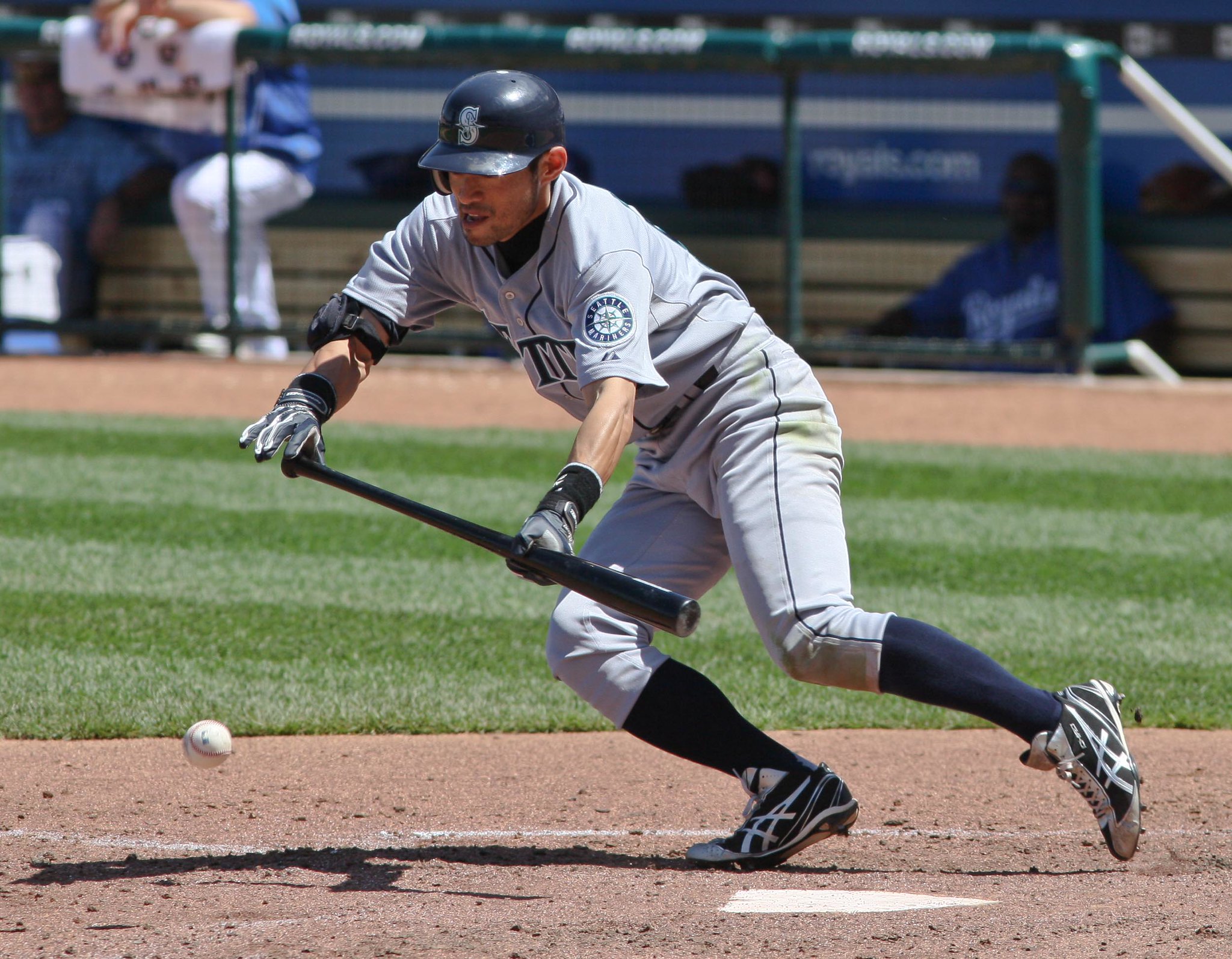In this image, a Japanese baseball player, likely from the Seattle Mariners, is captured in the process of laying down a bunt at home plate. He is wearing a gray uniform with "Seattle" emblazoned on it, paired with blue socks and cleats that appear to be Asics brand. The player, a left-handed batter, is positioned with his bat held horizontally in front of him, gripping it with his left hand at the edge and his right hand in the middle, indicative of a bunting motion. He sports a dark blue helmet featuring a protective covering around his right ear, which has an "S" on the front, and a black elbow pad on his right elbow along with batting gloves. In the background, home plate, the ball lying in front of him, and the dirt of the field are visible, along with a fence behind the home plate area. Beyond the fence, the dugout is visible with some players seated, and a patch of grass separates the batter from the dugout.